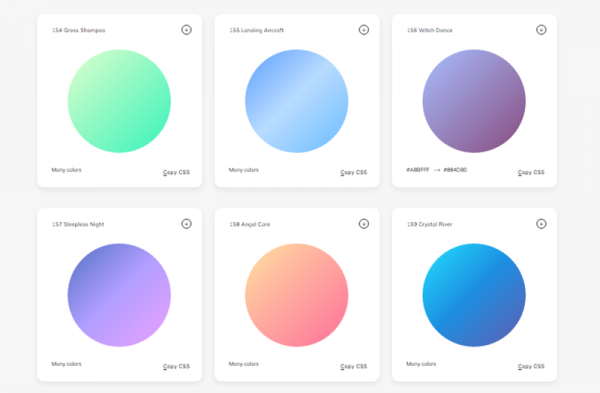A detailed screenshot displays an array of colored balls organized into two rows, set against a clean, minimalistic background. Each ball is positioned within a square, and the bottom corner of each square features text indicating either "CCS" or "CSS."

In the first row, from left to right, there is a green circle, a light blue circle, and a purple circle. Each of these circles exhibits a subtle shading effect where the bottom part of the circle is darker, gradually transitioning to a lighter shade towards the top.

In the second row, from left to right, there is a bluish-purple circle, a pink circle, and a blue circle. The bluish-purple and blue circles also showcase a gradient shading, but in reverse order compared to the first row: they are darker on the top and become lighter towards the bottom. The pink circle follows the same shading pattern as the purple and blue circles in this row.